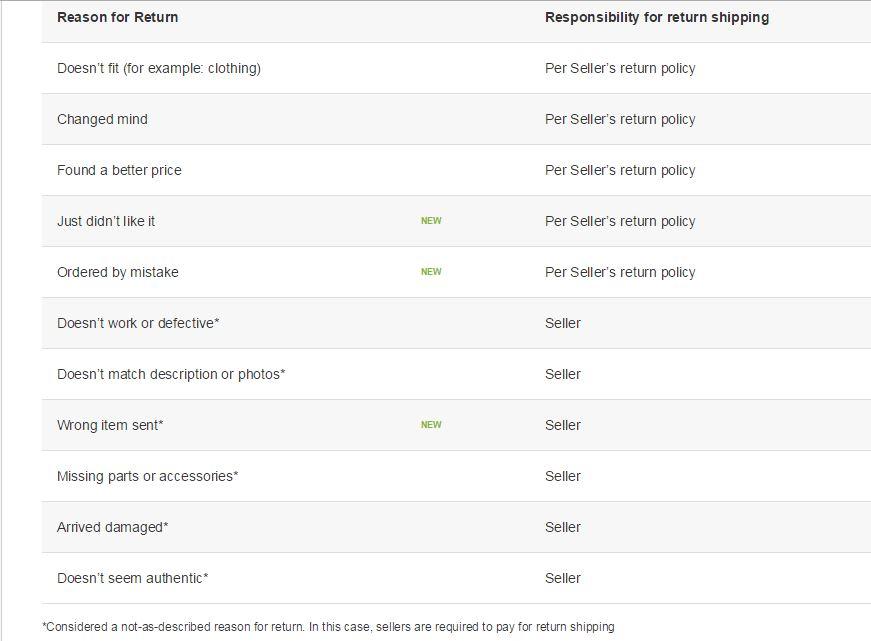**Screenshot of Return Window on E-commerce Website**

In the upper left corner, bold black letters state "Reason for Return," while across on the right, bold black letters spell out "Responsibility for Return Shipping." The rest of the text is in regular black letters.

On the left side of the screen, under "Reason for Return":
- Doesn't fit (e.g., clothing)
- Changed mind
- Found a better price
- Just didn't like it
- Ordered by mistake
- Doesn't work or defective *
- Doesn't match description or photos *
- Wrong item sent *
- Missing parts or accessories *
- Arrived damaged *
- Doesn't seem authentic *

A note at the bottom explains that reasons marked with an asterisk (*) are considered "Not as Described" reasons for returns. In these cases, sellers are required to pay for return shipping.

In the middle column, the text "per seller's return policy" appears five times in green letters.

On the right side, under "Responsibility for Return Shipping":
- Per seller's return policy (repeated five times)
- Seller